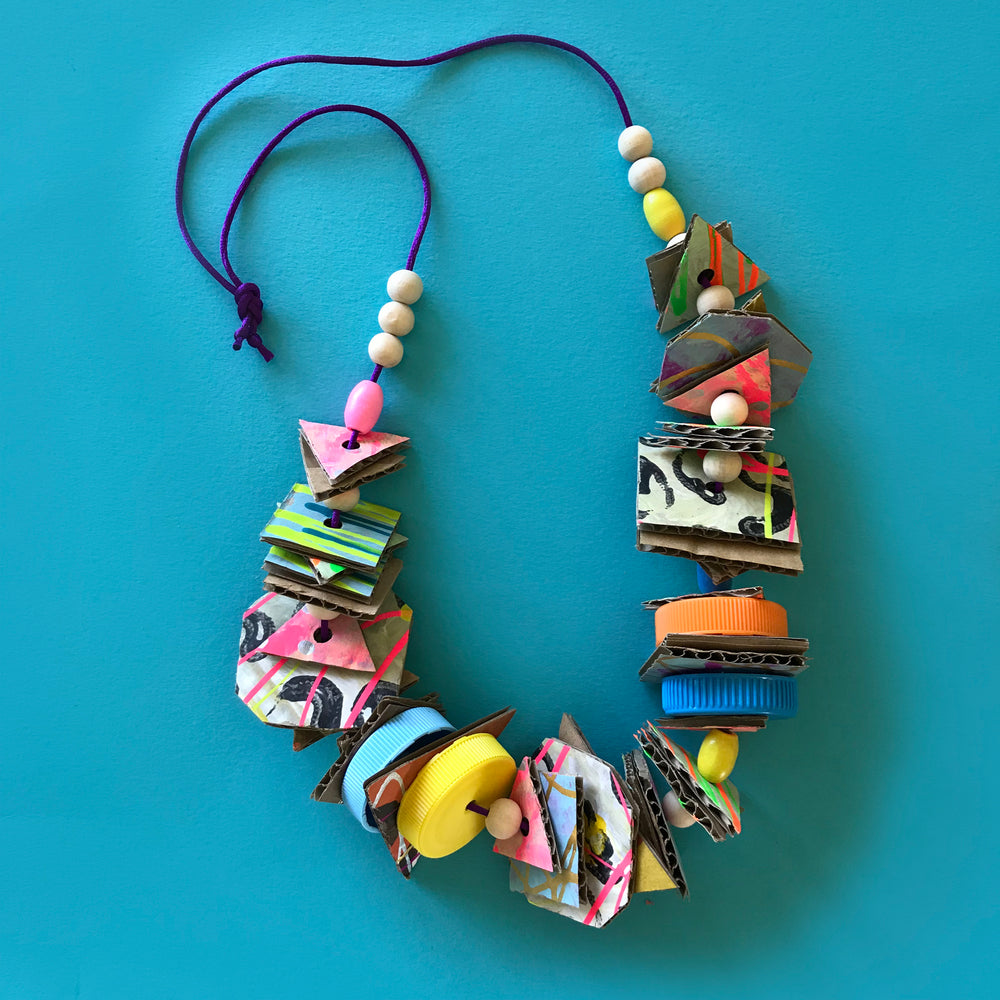The image captures a necklace crafted from an eclectic mix of materials, laid out on a teal, rectangular background. The necklace is held together by a cord that appears to be a royal blue or purplish-blue color, tied at the top. This homemade adornment features an array of vibrant items: multicolored bottle caps in shades of orange, blue, yellow, and light blue; white, pink, and yellow beads interspersed throughout; and various shapes cut from thick cardboard, including triangles and squares. These cardboard shapes are painted in a medley of bright colors, adding to the necklace's lively aesthetic. Some shapes even appear to have a spray-painted effect, with colors like red, black, and green. The overall arrangement is reminiscent of something exuberant and whimsical, perhaps akin to 1980s or 1990s pop culture fashion.